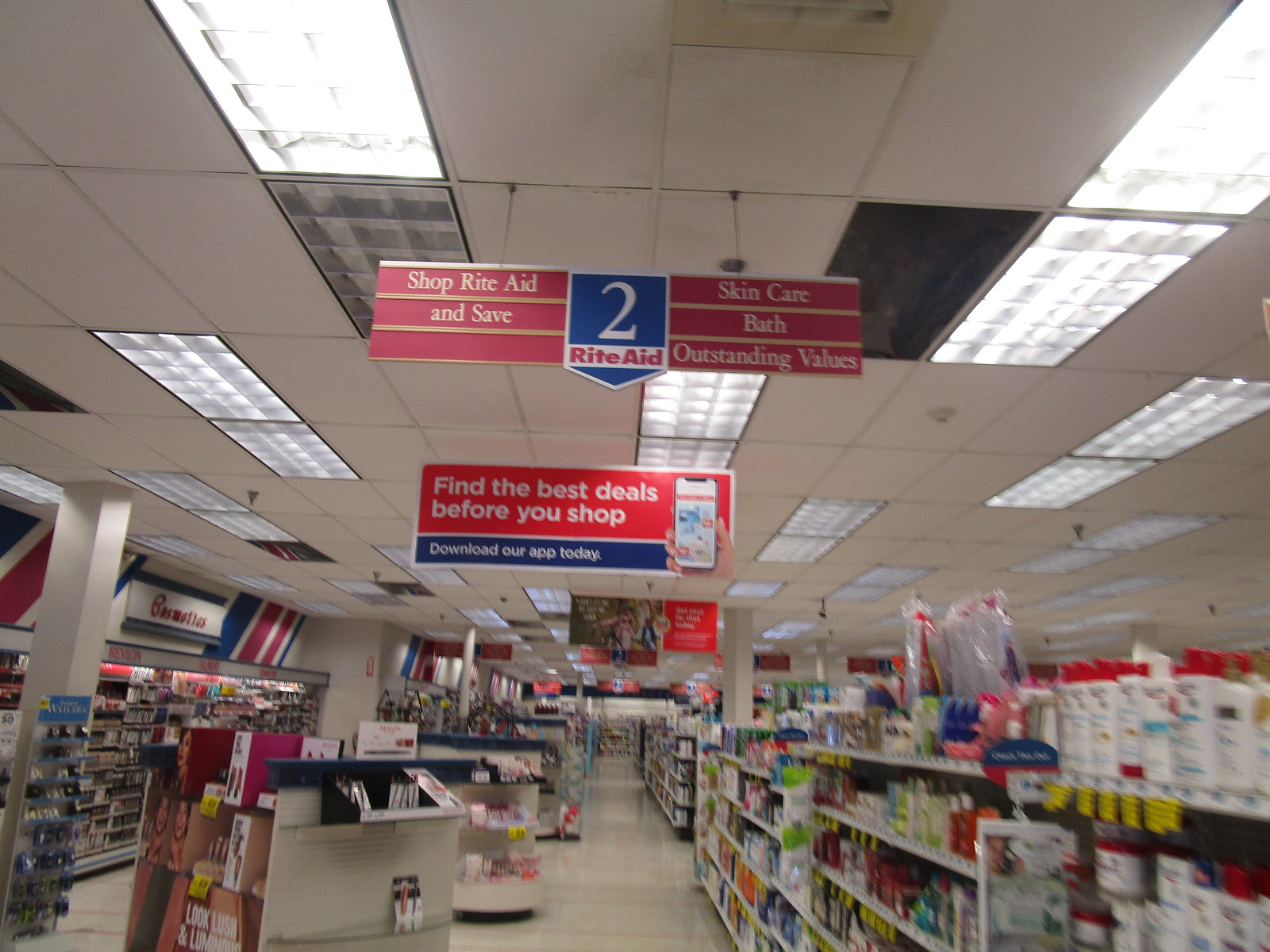This is a color photograph of the interior of a Rite Aid store, specifically showing aisle number 2. The camera is angled slightly upwards, capturing a white paneled ceiling with large rectangular lights. Hanging from the ceiling is a prominent sign that reads "Shop Rite Aid and Save" with specific mentions of "Skincare," "Bath," and "Outstanding Values." The sign also displays a blue section with the words "Rite Aid" and the aisle number "2." Below, shelves are stocked with various products, including cosmetics and skincare items. On the left, there's another sign denoting cosmetic brands. Additionally, standalone racks holding makeup products are visible in the center, along with shelves on the right filled with various goods. Further down the aisle, another banner reads "Find the Best Deals Before You Shop. Download Our App Today," accompanied by an image of a phone. There's a third sign in the background, slightly blurry and difficult to read, but it appears to feature an image of a child. The polished white floor reflects the overhead lighting, adding to the store's bright and clean appearance. The photograph is slightly blurry near the front, but it clearly captures the store's organized layout and promotional signage.